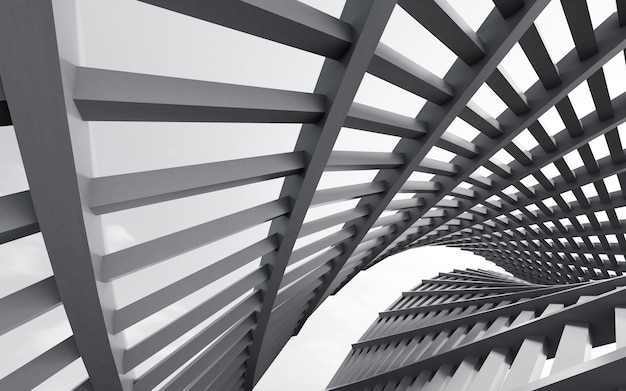The image depicts a meticulously crafted piece of digital artwork, showcasing a warped metal fence or gate reminiscent of a prison door. The gate, composed of vertical and horizontal gray metal bars, twists and curves in an unnatural manner, suggesting the use of CGI or computer-generated imagery. The structure, which begins on the left side of the image with a segment that curves backward, appears to be observed from below, enhancing the dramatic effect of its bends and twists. The background features monochromatic hues of white and gray, likely representing the sky, and the entire scene is devoid of any other colors or textual elements. As the bars curve, the lines intersect, creating a pattern of longer lines transforming into small squares, embodying an abstract, modern, and minimalist aesthetic.